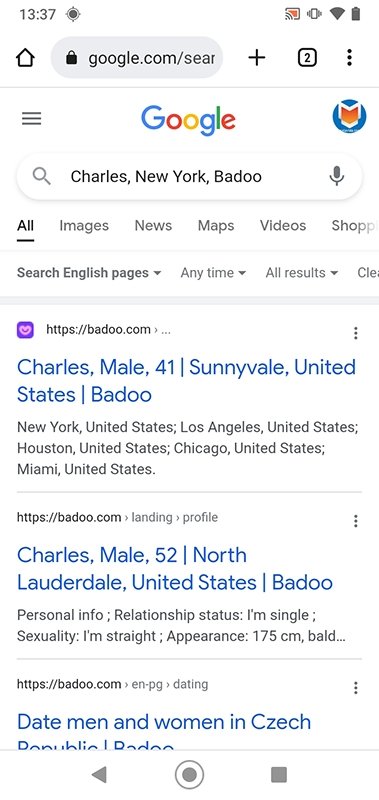**Screenshot of Web Search Results for "Charles, New York, Badu"**

The screenshot captures a web search made on Google for the terms "Charles, New York, Badu." The search results predominantly feature links to profiles and pages from the dating website Badu.com. Below is a detailed description of the content displayed in the search results:

1. **First Search Result:**
   - **Website:** Badu.com
   - **Profile Summary:** Charles, Male, 41, Sunnyvale, United States.
   - **Additional Locations Listed:** New York, United States; Los Angeles, United States; Houston, United States; Chicago, United States; Miami, United States.

2. **Second Search Result:**
   - **Website:** Badu.com
   - **Profile Summary:** Charles, Male, 52, North Lauderdale, United States.
   - **Personal Information:**
      - **Relationship Status:** Single
      - **Sexuality:** Straight
      - **Appearance:** 175 centimeters tall, bald

3. **Third Search Result:**
   - **Website:** Badu.com
   - **Link Description:** EN-PG > Dating
   - **Content:** Date men and women in the Czech Republic on Badu.com

Overall, the search results highlight profiles named Charles from various locations in the United States, as well as a general dating page for the Czech Republic on Badu.com.